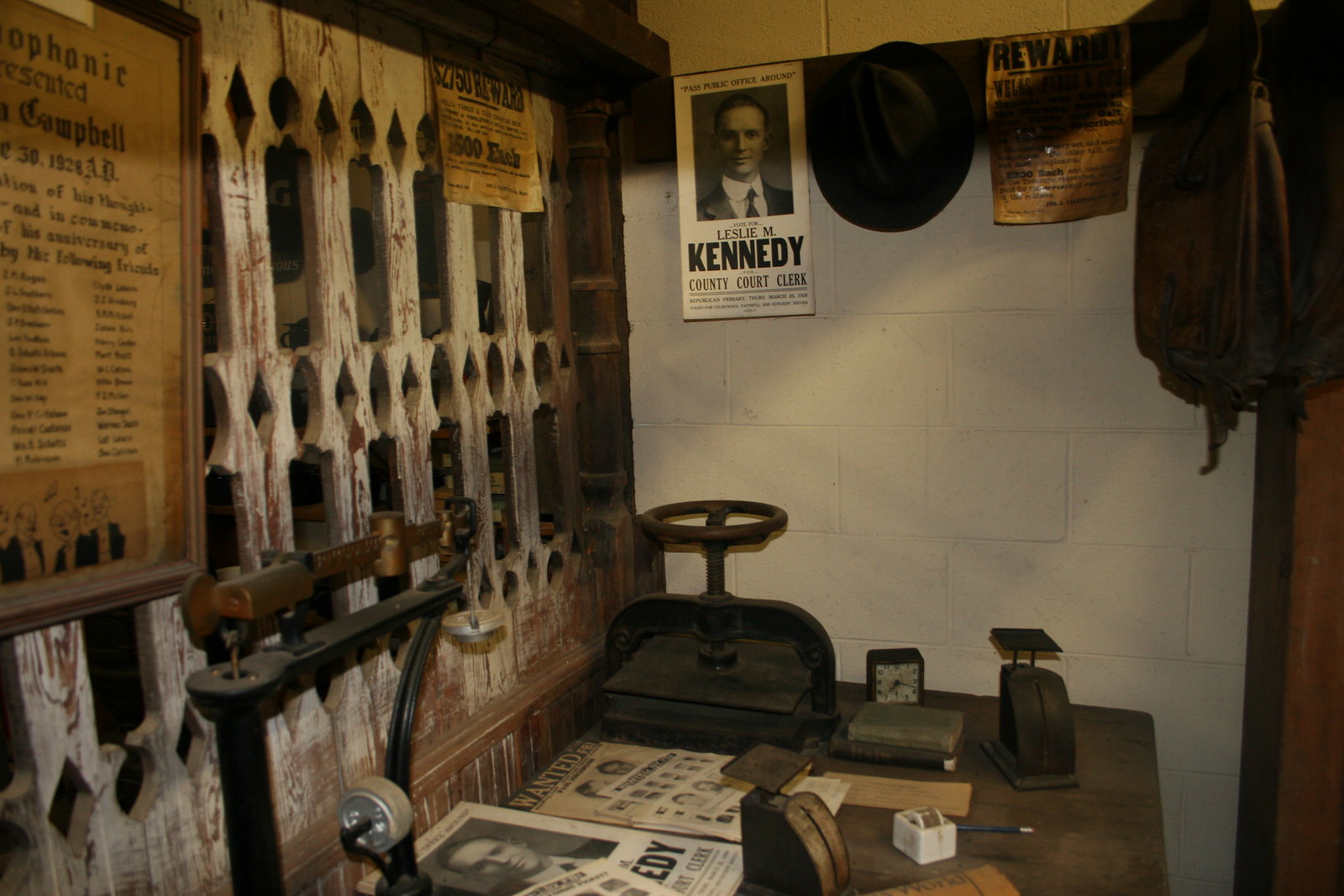This image appears to be taken inside a historical museum or a vintage-themed display area, showcasing an eclectic collection of antique items. Dominating the left side of the picture is an old picket fence with worn white paint, indicative of its age. In the foreground, a cluttered desk is strewn with black and white photos, an old clock, and what seems to be a set of balancing scales. Various metal apparatuses and machinery, perhaps a press or a vice with a wheel on top, are visible, adding to the historical feel of the room.

The walls are adorned with numerous posters, prints, and signs. Notably, there's a political poster reading "Leslie M. Kennedy for County Court Clerk," which might suggest the era of the 1930s. Accompanying this are FBI wanted posters and a reward notice offering a $2,750 reward, hinting at the law enforcement theme prevalent in the display. An old fedora hat hangs on a hook, further enhancing the vintage ambiance.

The setting is mostly monochromatic, with a mixture of white and black tones dominating the objects and the walls. The white walls, paired with a brick section and wooden framing, add depth to the scenery, making it reminiscent of a police station or a historical archive, complete with evocative memorabilia of a bygone era.